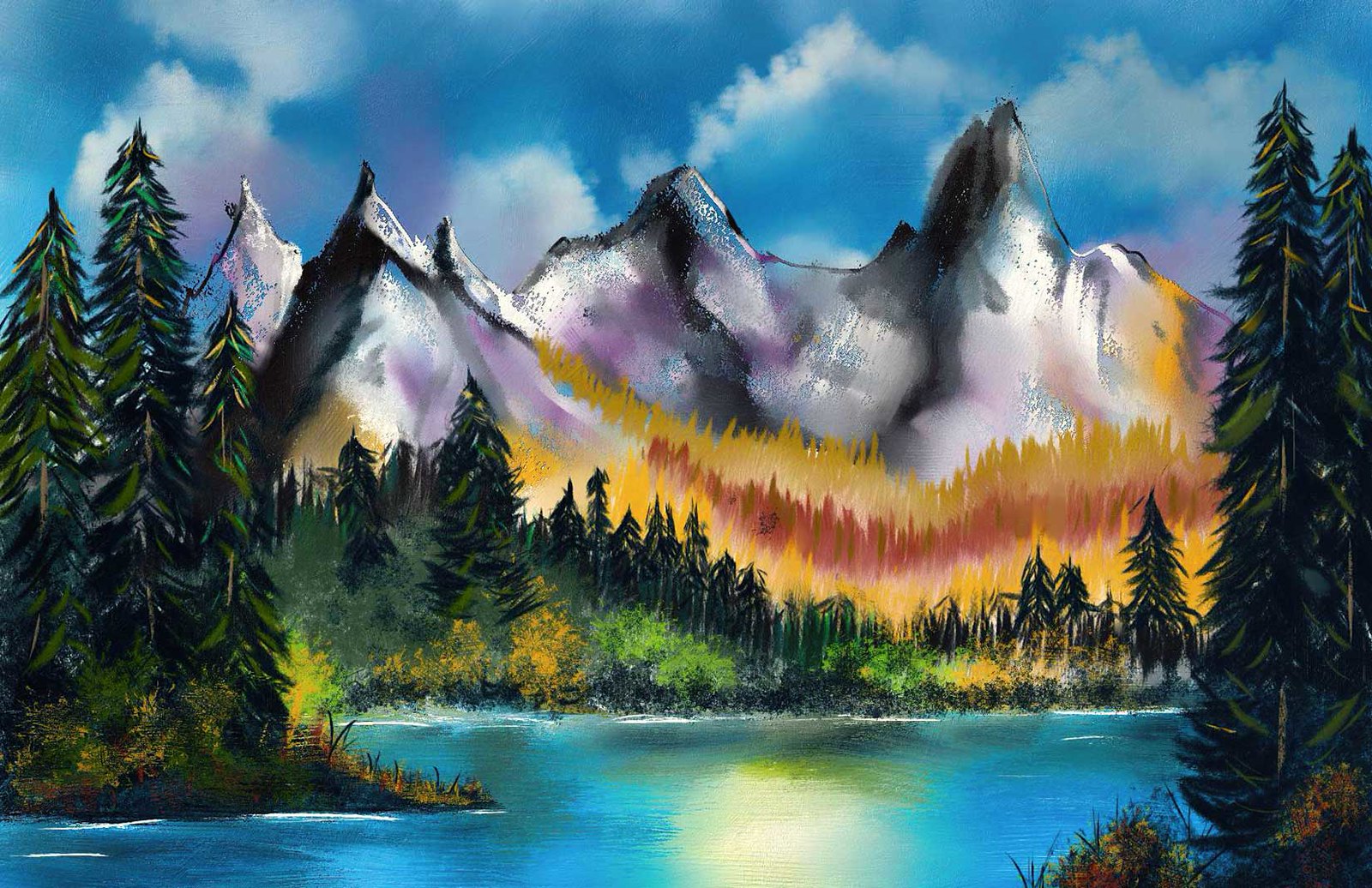The image is an intricately detailed nature painting, seemingly created in oil, capturing a serene outdoor scene. In the foreground lies a tranquil blue lake, its surface reflecting shadows and light from the sky above, as well as the tree line that encircles the water. The left side of the painting features a small hill jutting into the lake, adorned with tall, slender, and pointy pine trees, their bases enveloped in lush greenery and bushy foliage. The right corner shares a similar composition, with two more towering pine trees rising from a patch of shrubs, their tips adorned with an orange hue, suggesting blooming flowers.

The background is dominated by jagged, sharp-tipped mountains, painted in shades of grayish-purple and white, indicating snow cover. These mountains rise majestically into a medium blue sky dotted with fluffy white clouds. Transitioning from the mountains to the lake below is a gradient of trees, from the tall, skinny pines to smaller, rounder trees dressed in autumnal colors of yellow, orange, and red. The entire scene conveys a sense of peacefulness and natural beauty, encapsulated in the harmonious blend of colors and textures.